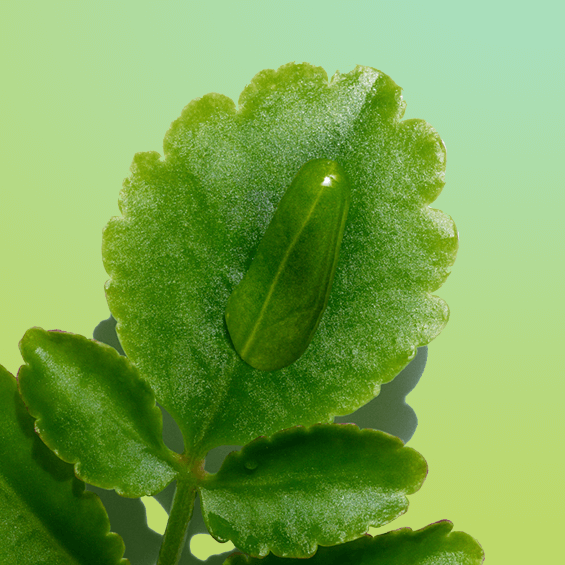The image is a close-up of a plant showcasing a large leaf with scalloped edges and a rough surface due to small indentations. This main leaf, occupying a significant portion of the image, holds a large, oval-shaped droplet of water which magnifies the veins and reflects a hint of sunlight. The leaf appears to have white specks, possibly frost, that the water has melted away, revealing the leaf's textured surface. Below the main leaf, a stem runs from the bottom left to the right, supporting two smaller leaves: one extending to the left and the other straight to the right. These smaller leaves share the rough texture of the larger leaf. Behind the plant, there is a light greenish background that fades to gray in some areas, with a faint shadow of the plant cast upon it. Additional, partially visible leaves extend off the page from the bottom left. The overall composition of the image highlights the intricate details and textures of the plant, set against a soft, unevenly lit background.